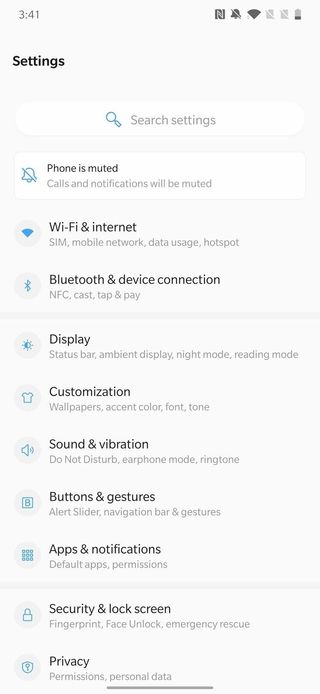The screenshot depicts a phone's settings menu. At the top, the word "Settings" is prominently displayed. Directly below it, there is a search bar featuring a blue magnifying glass icon, allowing users to search within the settings. The settings are organized into several rows, each representing different options.

The first option indicates that the phone is currently muted, giving users the ability to mute or unmute the device. The subsequent settings include:

1. **Wi-Fi & Internet:** Represented by a blue wedge icon.
2. **Bluetooth & Device Connection**

Following this, the settings options continue with:
3. **Display:** Illustrated by a half-colored sun icon with emanating lines.
4. **Customization**
5. **Sound & Vibration**
6. **Buttons & Gestures**
7. **Apps & Notifications**
8. **Security & Lock Screen**
9. **Privacy:** Positioned at the very bottom of the list.

Each setting is accompanied by a small graphic icon that visually represents the specific function, enhancing the intuitive navigation of the menu.